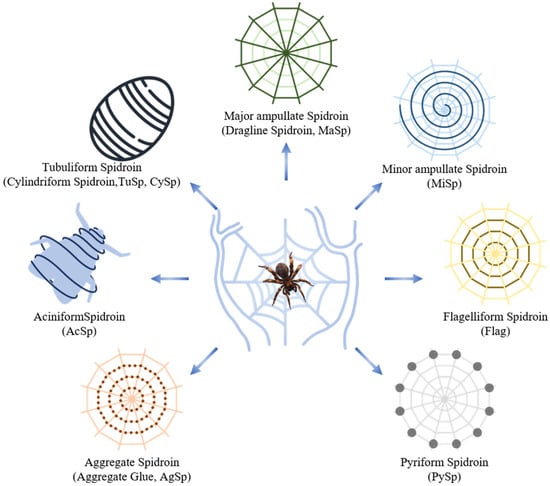This is a detailed scientific diagram depicting various types of spider webs and the proteins associated with their construction. At the center of the image, a brown spider, resembling a tarantula or brown recluse, is positioned head-down within a blue web featuring some internal bracing structures or branches. Surrounding this central illustration are seven blue arrows radiating outward, each pointing to different line drawings of spider webs, labeled with their respective spidroin types.

1. At the top center, there is a major ampullate spidroin web, resembling a Ferris wheel with concentric rings.
2. To the upper right, a minor ampullate spidroin web is illustrated with a spiral design leading towards its center.
3. Further down on the right, a flagelliform spidroin web is depicted with a tan and brown dream-catcher-like structure.
4. At the bottom right, a piriform spidroin web has several gray dots along its perimeter.
5. Moving clockwise to the bottom left, a tubuliform spidroin web is shown as a striped, egg-shaped figure.
6. Above this, an aciniform spidroin diagram features an insect-like figure wrapped in a spiral pattern.
7. To the upper left, an aggregate spidroin web is characterized by its dot-based spiral, shown in mauve, and brown tones.

The diagram provides a comprehensive visual guide to understanding the different web structures produced by spiders, emphasizing the intricate and varied nature of their silk proteins.